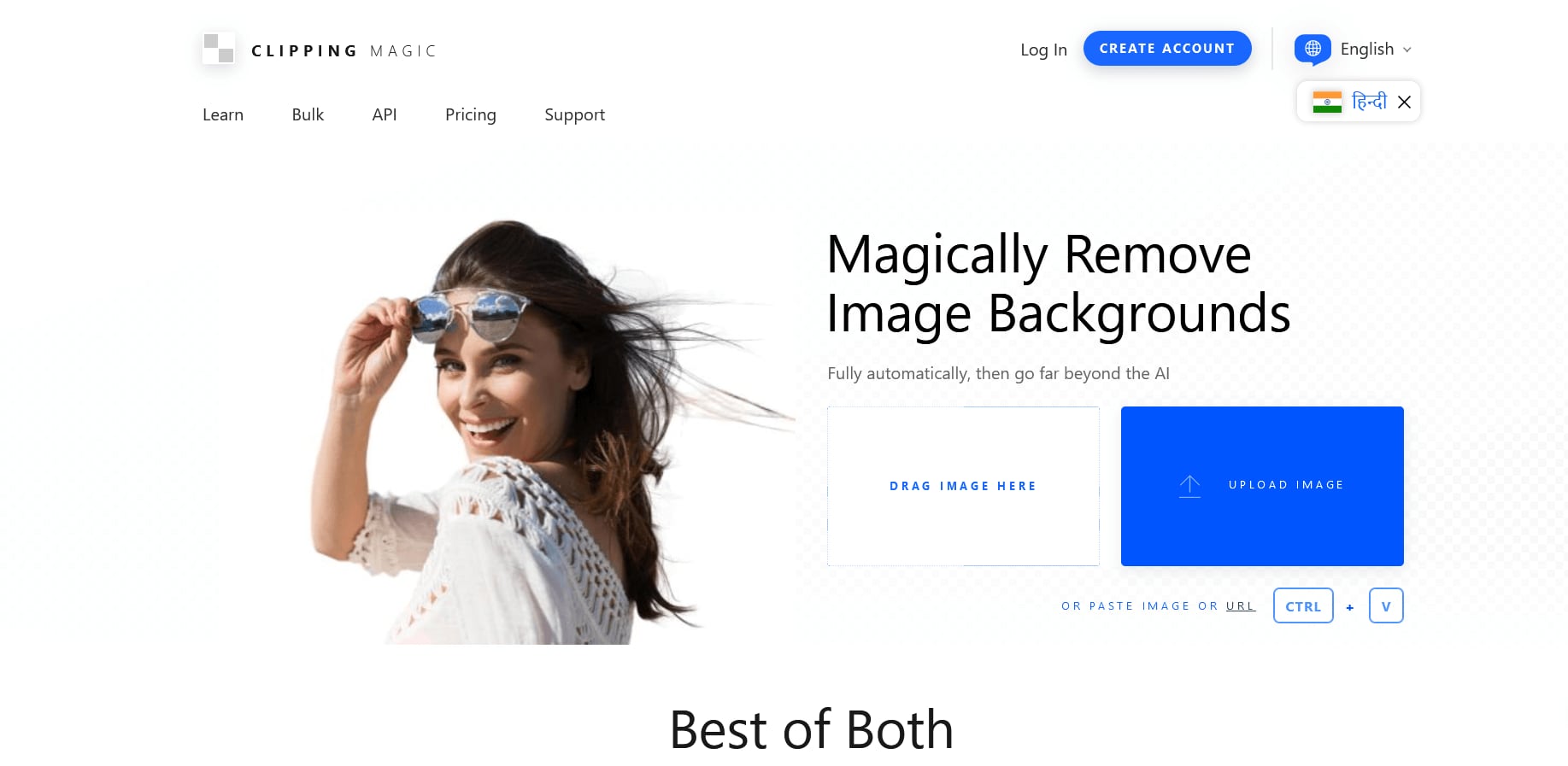The screenshot displays a vibrant and user-friendly website interface. In the upper left corner, there is a small square containing the "Clipping Magic" logo, represented by two black squares. On the upper right, the navigation features prominently with a "Login" button and a "Create Account" button, both in blue, accompanied by a language selection drop-down set to English.

The centerpiece of the screenshot is a striking, colorful image of a young, attractive woman captured from mid-back up. She faces west, her body slightly turned forward, revealing her long brown hair cascading down. With her right hand, she lifts a pair of sunglasses just above her eye, adding a casual and stylish touch to her appearance. She is dressed in a white crocheted shirt, enhancing the overall appeal.

To the right of her image, enticing text reads: "Magically remove image backgrounds, fully automatically, then go far beyond the AI." Below this text, two buttons invite user interaction: a white button with blue text labeled "Drag Image Here," and a blue button with white text labeled "Upload Image." Further beneath these buttons, instructions appear: "Or paste image or URL." This interface suggests a seamless and advanced tool for automatic image background removal and editing.